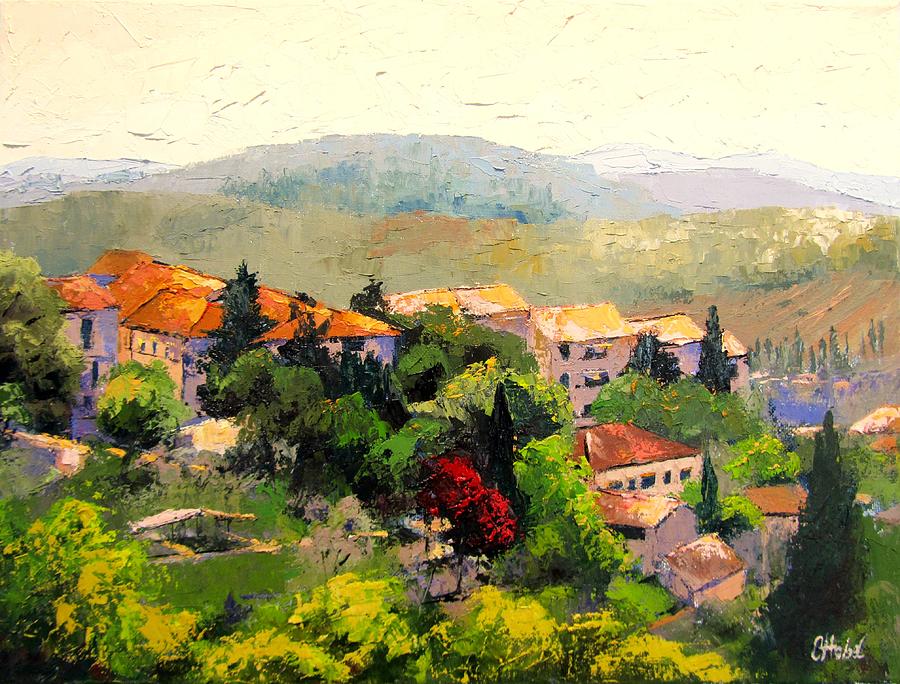This impressionistic painting captures a picturesque European village nestled on a lush, green mountainside. The scene is dotted with houses featuring white sidings and warm-hued roofs that range from orange and yellow to red. Trees with predominantly green foliage, along with a couple of trees showcasing vibrant red leaves, are interspersed among the houses. A subtle water feature appears on the right side of the image, adding a tranquil element to the composition.

In the background, an array of gray and white mountains rise majestically, suggesting a distant forest or further hilly terrain beneath a tan-colored sky. The brush strokes of the thick oil paint are messy and slightly abstract, characteristic of the impressionistic style, lending a soft, almost dreamy quality to the overall scene. 

The painting is rectangular, with the longer sides at the top and bottom, creating a broad landscape view. Finally, the artist's signature, appearing to start with the letters "CH," is inscribed in the lower right-hand corner. The slightly peeling appearance of the paint adds a vintage charm, making this an evocative depiction of a serene, timeless village.